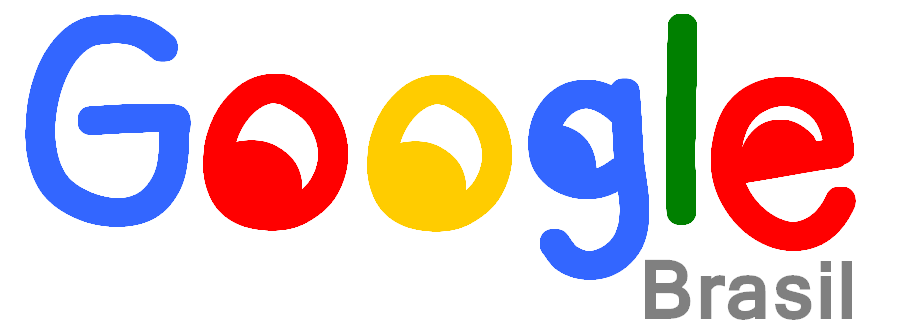The image features a hand-drawn style version of the Google logo against a white background. The letters in "Google" appear in varying vibrant colors: a blue capital 'G', a red lowercase 'o' with a small red dot resembling an iris pointing to the left, a yellow lowercase 'o' with a corresponding yellow dot also looking left, a blue lowercase 'g' with a similar pupil effect, a green 'l', and a red 'e' with an iris facing directly forward. Below the logo, in smaller gray print, is the word "BRASIL" (spelled with an 'S', not a 'Z'). The pupils within the letters give the impression of eyeballs looking in different directions, adding a playful touch to the artwork.